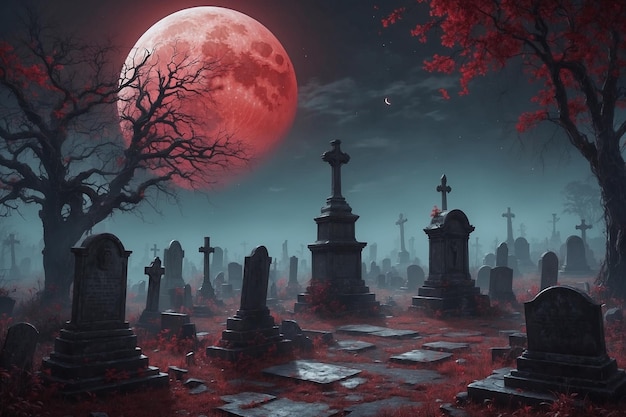This atmospheric artist’s rendering depicts a densely packed cemetery at night, illuminated by an unnaturally large, glowing pinkish-red moon dominating the upper left corner of the sky, alongside a tiny crescent moon-like object. The graveyard is crowded with a plethora of grayish headstones, many adorned with crosses or domed tops, hinting at their aged and slightly askew positions. Both upright headstones and flat graves are present, set against an eerie backdrop of craggly, mostly bare trees with a few ominous reddish leaves. Red foliage covers the ground, interspersed with a lingering night fog that enhances the scene's haunting ambiance. Inlaid stone pathways navigate through the chaotic array of gravestones, reinforcing the impression of a long-forgotten, overgrown resting place. The sky casts a bluish-green-gray hue, further immersing the viewer in the cool, eerie atmosphere of a fall night.